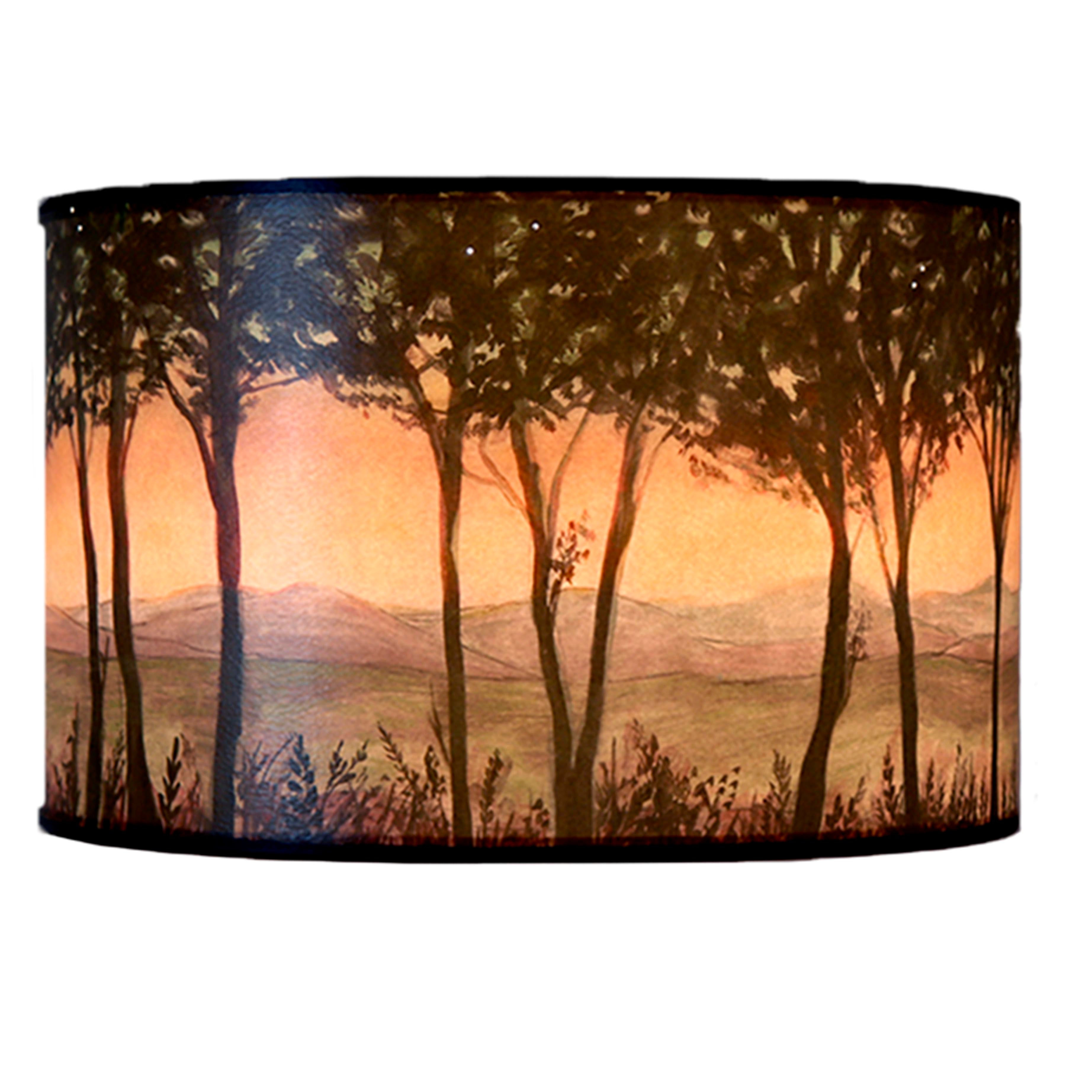The image showcases a drum lampshade adorned with a loose, artistic painting of a woodland scene. The design features narrow tree trunks and limbs extending from a grassy knoll at the base to a leafy canopy at the top. The scene captures a mountainous background with a warm, orange-tinted sky, suggesting a sunset filtering through the trees. Predominantly earth tones of browns, reds, oranges, and greens create a cohesive, warm palette. The painting's details are not sharp but rather have a fluid, interpretive quality. The lampshade itself has black borders at the top and bottom, and the image appears to be placed against a plain white background, likely for a product photo that emphasizes the item without distractions. The entire artwork on the round lampshade is intended to be illuminated from within, enhancing the vibrancy of the colors and the depth of the scene.